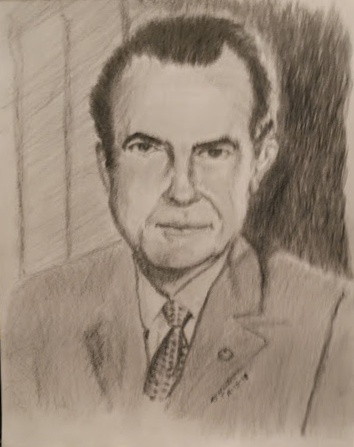This image showcases a detailed pencil sketch of an older man drawn from the chest up, centered in a portrait-style composition. The edges of the paper are not visible, giving the impression that we are looking straight at the artwork. The man, whose identity isn't immediately recognizable but gives an impression of familiarity, is depicted wearing a suit and tie. The artist has skillfully used varying pressures of the pencil to create contrasting light and dark areas, enriching the drawing with depth and texture. 

The man's short hair is neatly styled, his clean-shaven face accentuating the wrinkles around his mouth, which suggests his older age. His eyes are open, giving the portrait a contemplative and engaging expression. Defined eyebrows frame his eyes, contributing to the lifelike quality of the sketch. The background is intriguing, with a heavily shaded area to the right of the man and what appears to be a white picket fence on the left, which adds a subtle narrative element to the otherwise straightforward portrait.